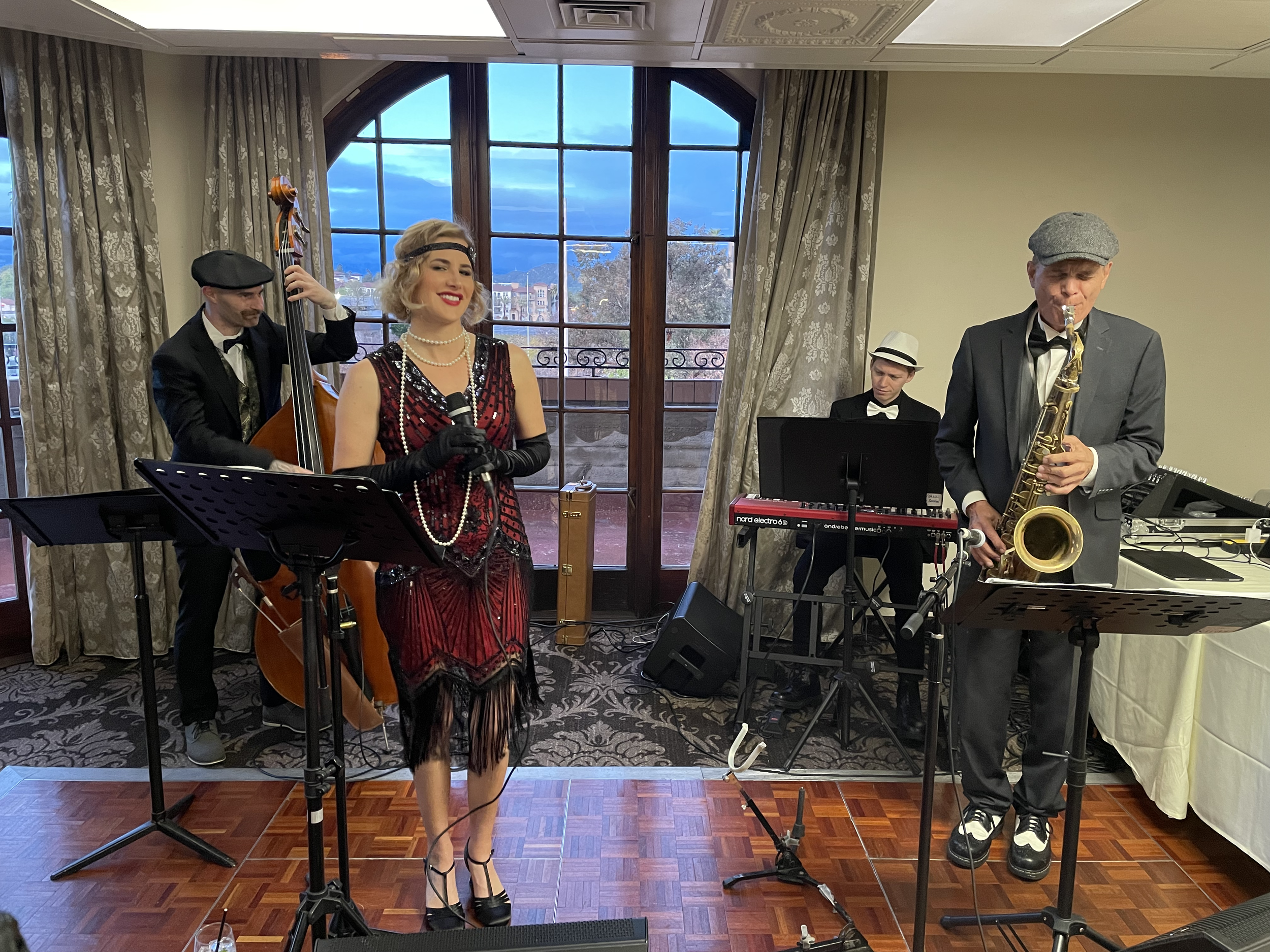The photograph depicts a four-piece band performing in a well-lit room with large windows offering a stunning view of a sprawling cityscape under a blue sky. Beige walls and gray curtains with white detailing frame the image. On the far left, a man stands playing a stand-up bass. He wears a black suit with a white shirt, black bow tie, and a greenish vest, along with a black hat and gray dress shoes. To his right, a woman dressed in a red flapper dress with black fringe at knee-level stands holding a microphone. She has short blonde hair adorned with a black headband, dark eyebrows, red lipstick, long pearl necklaces, and elbow-length black gloves. Her black heels peek out from under her dress. Next to her, a man sits at a red electric keyboard. He wears a black suit with a black shirt, a white bow tie, and a white fedora with a black band. On the far right, an older gentleman plays a saxophone. He wears a gray suit with a white collared shirt, a black bow tie, white and black wingtip shoes, and a gray newsboy cap. All musicians have music stands in front of them, and they are situated on a floor that transitions from shiny wood to a carpet with a white floral pattern. White tables are visible to the right, perhaps moved aside to accommodate the performance. The overall ambiance suggests an elegant event, possibly in a hotel ballroom or a similar upscale venue.